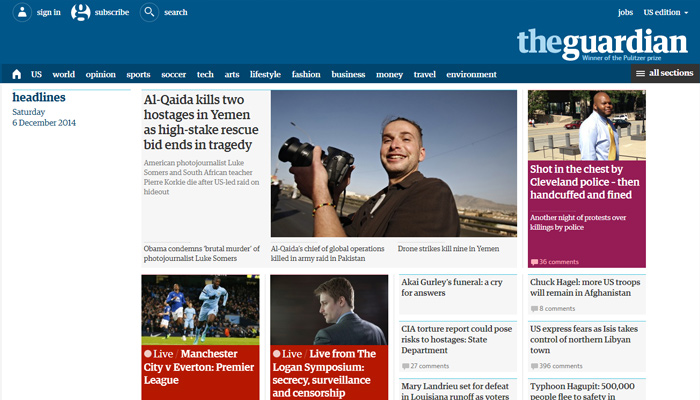This image, sourced from The Guardian's website, showcases the detailed layout of its homepage. At the top right corner, the site's branding is prominent with 'The Guardian' banner, which features the name in white against a light blue background. The branding is encapsulated as a single word, positioned in the top left corner alongside navigation options for signing in, subscribing, and searching. Above the banner, there's an additional menu offering job listings and a US edition selector with a dropdown arrow for further options. Directly below the main banner, another navigation menu is visible, presenting sections such as US, World, Opinion, Sports, Soccer, Tech, Arts, Lifestyle, Fashion, Business, Money, Travel, and Environment. A brown box labeled 'All Sections' provides access to further content categories.

The main portion of the homepage is dedicated to showcasing various articles. The leading article, highlighted prominently, reports on a tragic event: "Al Qaeda kills two hostages in Yemen as high-stake rescue bid ends in tragedy." Surrounding this main article are other news stories, providing a comprehensive overview of the latest updates and diverse topics covered by The Guardian.